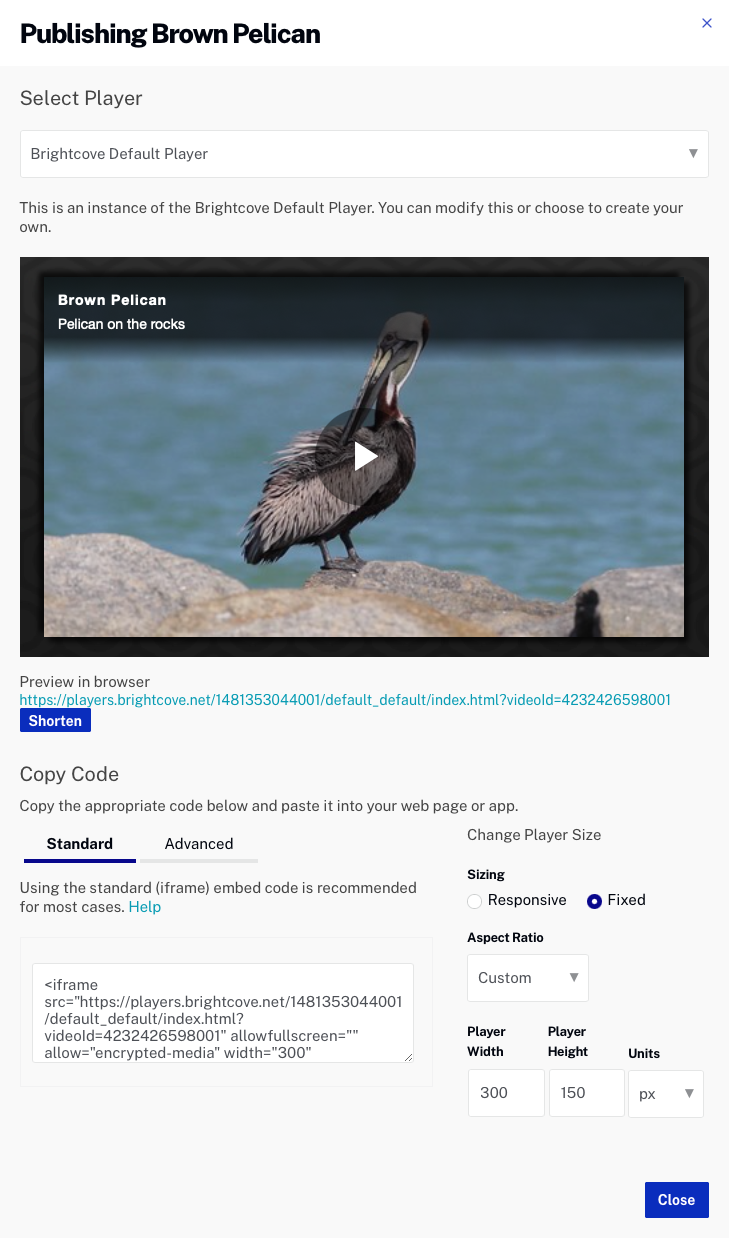Screenshot of a video player interface featuring a brown pelican:

The screenshot captures a webpage displaying a video interface. At the top left corner, the text "Publishing Brown Pelican" is visible. Directly below this, there is an option labeled "Select Player," allowing users to choose their preferred video player. In this instance, the "Brightcove Default Player" has been selected. A message underneath states, "This is an instance of the Brightcove Default Player. You can modify this or choose to create your own."

The thumbnail preview of the video, titled "Pelican on the Rocks," prominently features a brown pelican perched on gray rocks with the blue ocean in the background, indicating sunny weather. The pelican is depicted with its head bent backward, as if pecking at its feathers.

Below the video's thumbnail, there is a "Preview in Browser" link accompanied by a URL that users can copy to view the video in a web browser. Adjacent to this link is a purple button labeled "Shorten," which likely offers a function to condense the URL. Further down, there is a "Copy Code" button with corresponding video embed code displayed below it.